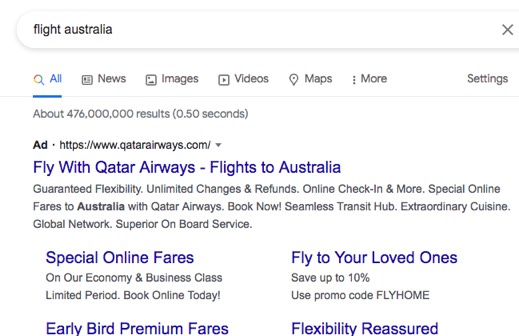The image displays a Google search results page with the query "flight Australia" entered in the search bar at the top left. Below the search bar is Google's menu array, featuring tabs labeled "All," "News," "Images," "Videos," "Maps," "More," and "Settings" from left to right. The search results indicate approximately 476 million results, returned in 0.50 seconds. The overall background is a clean white.

Under the search bar is an advertisement prominently highlighted with the text "Ad" in bold black letters. The URL displayed is "https://QatarAirways.com" and the linked blue text reads "Fly with Qatar Airways flights to Australia." The advertisement details various benefits including "Guaranteed flexibility, unlimited changes and refunds, online check-in, and more," and highlights "Special online fares to Australia with Qatar Airways." Additional features promoted include "Seamless transit hub, extraordinary cuisine, global network, and superior onboard service."

In a blue hyperlink, it mentions "Special online fares," followed by gray text explaining these are available for both economy and business class for a limited period, urging users to "Book online today." To the right, a promotion states "Fly to your loved ones, save up to 10%," with the promo code "FLIGHTHOME." To the left, there's mention of "Early reprieve fares" and at the bottom, a note ensures "Flexibility reassured."